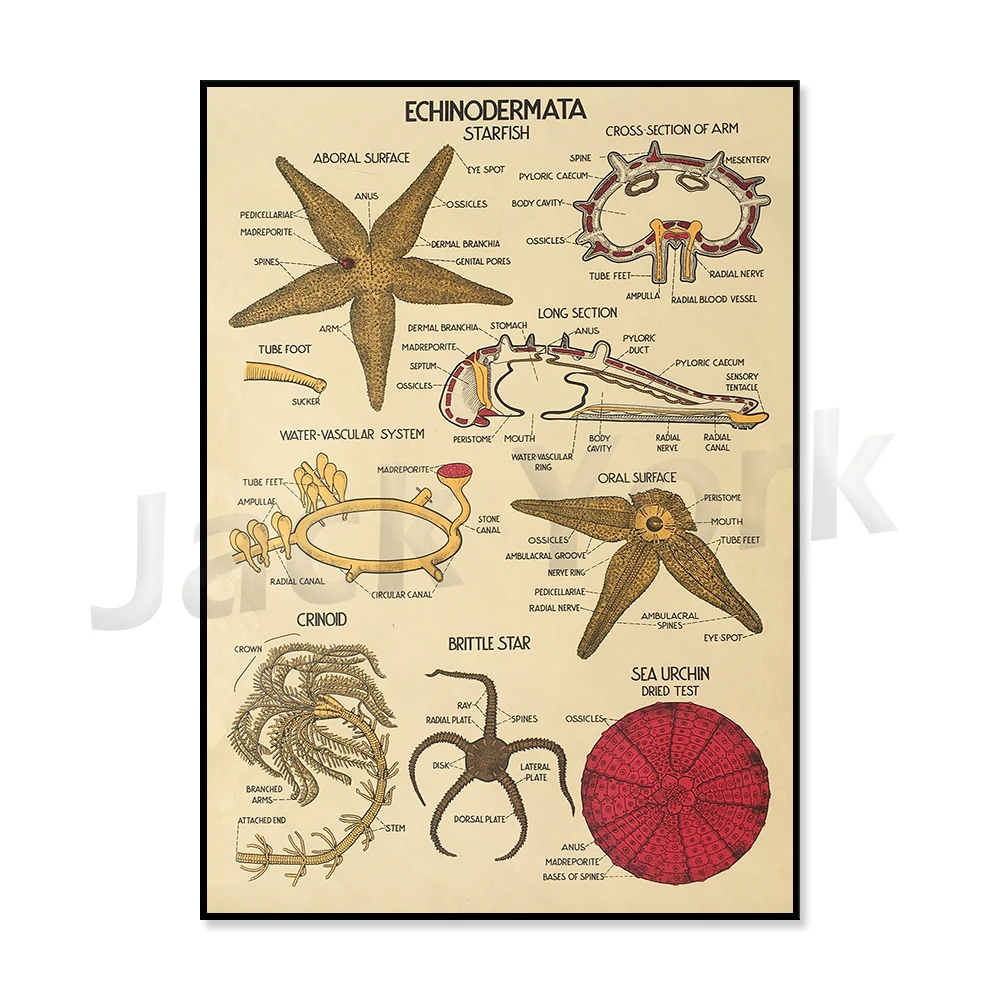The image is a detailed educational poster with a cream background and a black border, focused on the phylum Echinodermata, prominently featuring starfish and other sea organisms. At the top, the title "Echinodermata" is written in black, alongside an illustration of a brown starfish with dotted detail. Below the title, the poster presents various anatomical drawings of starfish, including a detailed cross-section of an arm showing grey and red cellular structure, a long section, a longitudinal section, and the water vascular system and oral surface.

The poster also depicts six to seven different sea organisms, mostly in shades of brown and yellow, with some variations such as a bright red sea urchin at the bottom right corner. Each organism is labeled with its scientific name, and their body parts are meticulously marked and described. The illustrations include the aboral surface of a starfish and a crinoid, which is characterized by its stem and branched crown, appearing more animal-like despite its plant-like appearance. Another significant illustration is of a brittle star, marked by its five slender and fragile arms. This comprehensive and detailed poster serves as an excellent educational tool to understand the diversity and anatomy of Echinodermata.